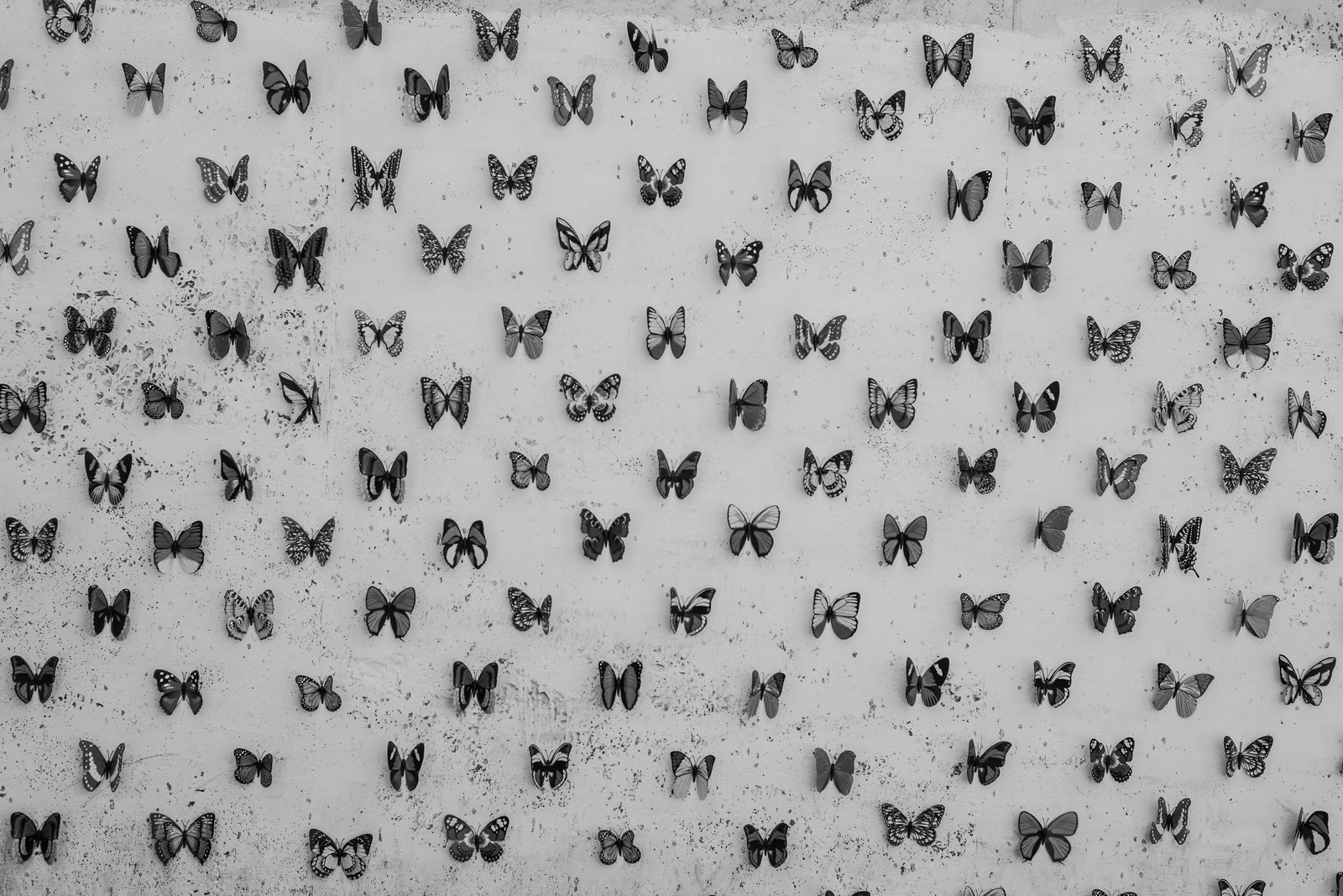The image is a black and white photograph depicting a display of various butterflies arranged neatly on a gray background that resembles a board or possibly a white pegboard. The butterflies, each with uniquely patterned wings, are meticulously pinned in staggered lines, ensuring they are evenly spaced apart. Their wings are flattened out to reveal intricate details, suggesting that this might be a collection from a butterfly enthusiast, possibly even a museum exhibit. The arrangement showcases a wide variety of butterfly species, highlighting the diversity within the collection.